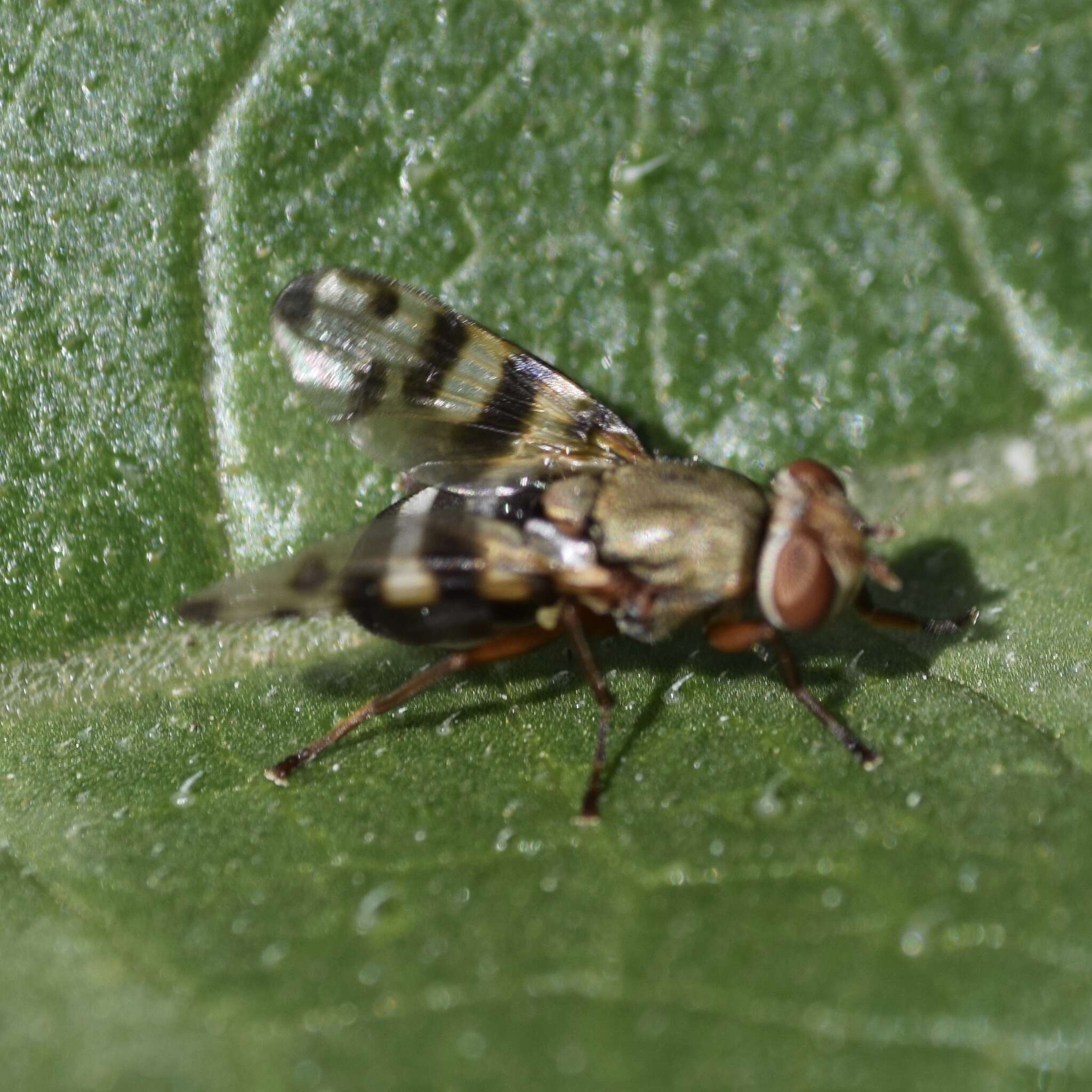This up-close photograph captures an insect perched on a leaf, presenting a detailed, side-profile view. The leaf, a dark green color mottled with white fuzz, reveals its veins and bumps. The insect, resembling a housefly or perhaps a bee, has a segmented black body with striking black and gold striped wings. Visible are four of its six legs, indicating its complex anatomy. The thorax is light brown, leading up to the head, which features large, distinctive, almost pinkish-brown eyes and prominent antennae. The photograph, while slightly out of focus, captures the insect in a moment of exploration, adding an element of dynamic curiosity to the image.